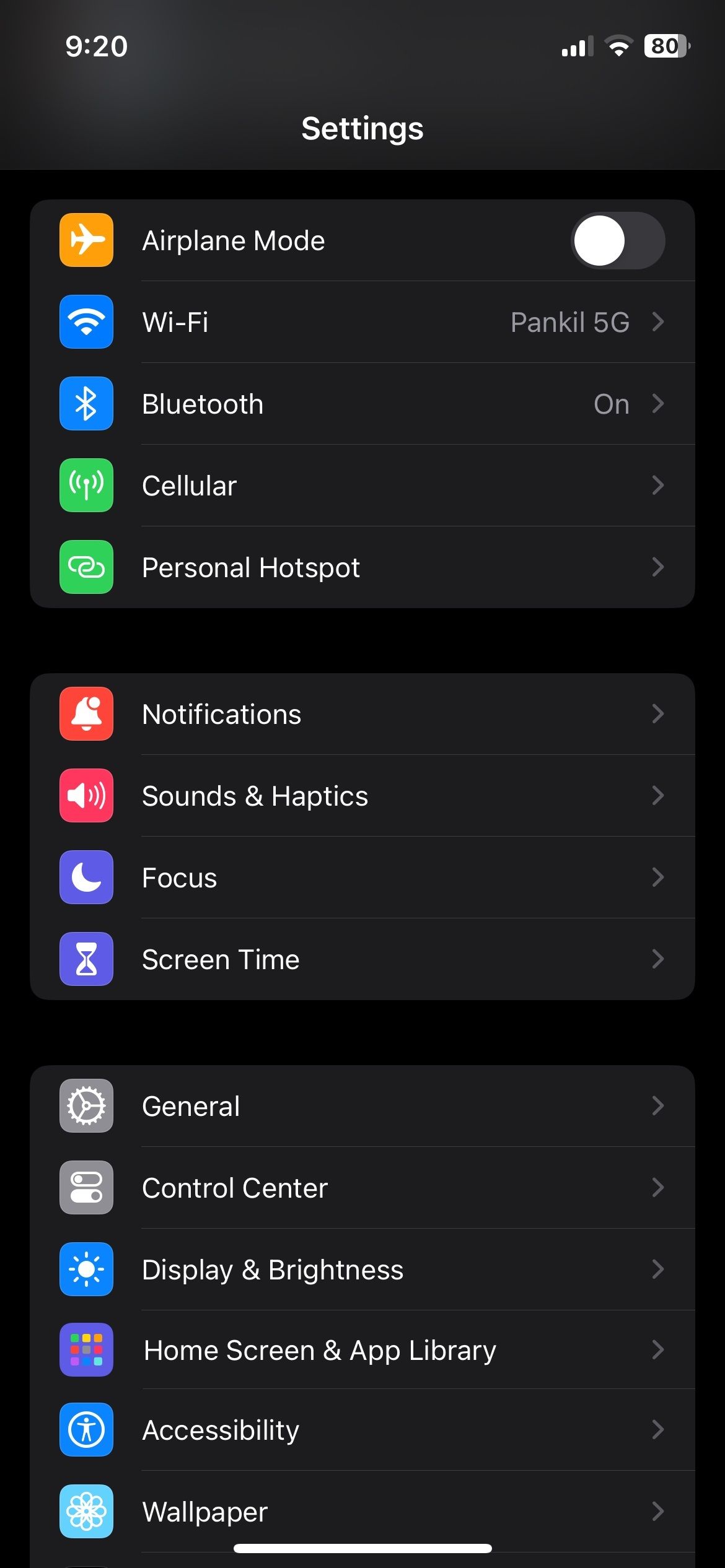The image is a screenshot of a cell phone screen, captured with the following details:

- **Top Bar:**
  - **Top Left Corner:** A black background with white text displaying the time "9:20."
  - **Top Right Corner:** Icons showing cellular connection, wireless signal, and battery status at 80%.

- **Main Content:**
  - **Header:** Centered text that reads "Settings."
  - **Menu Options:**
    - **Airplane Mode:** 
	  - Icon: Orange square with a white airplane.
	  - Status: Disabled
	- **Wi-Fi:** 
	  - Status: Connected to "Panko 5G"
	- **Bluetooth:** Enabled
	- **Cellular:** Listed
	- **Personal Hotspot:** Listed

	- **Notifications:**
	  - Icon: Red square with a white bell.
	- **Sound and Haptics:**
	  - Icon: Red square with a white microphone emitting sound waves.
	- **Focus:**
	  - Icon: Blue square with a white moon.
	- **Screen Time:**
	  - Icon: Blue square with an hourglass.
	- **General:**
	  - Icon: Gray square with a gear inside it.

	- **Control Center:**
	  - Icon: Gray square with an image inside it.
	- **Display & Brightness:**
	  - Icon: Blue square with an image of a sun.
	- **Home Screen & App Library:**
	  - Icon: Bluish-purple background with multicolored squares inside.
	- **Accessibility:**
	  - Icon: Blue square with a circle and a person inside it.
	- **Wallpaper:**
	  - Icon: Light blue square with an image.

Each option is accompanied by an intuitive icon that visually represents its function, providing a streamlined and navigable layout for managing various device settings.